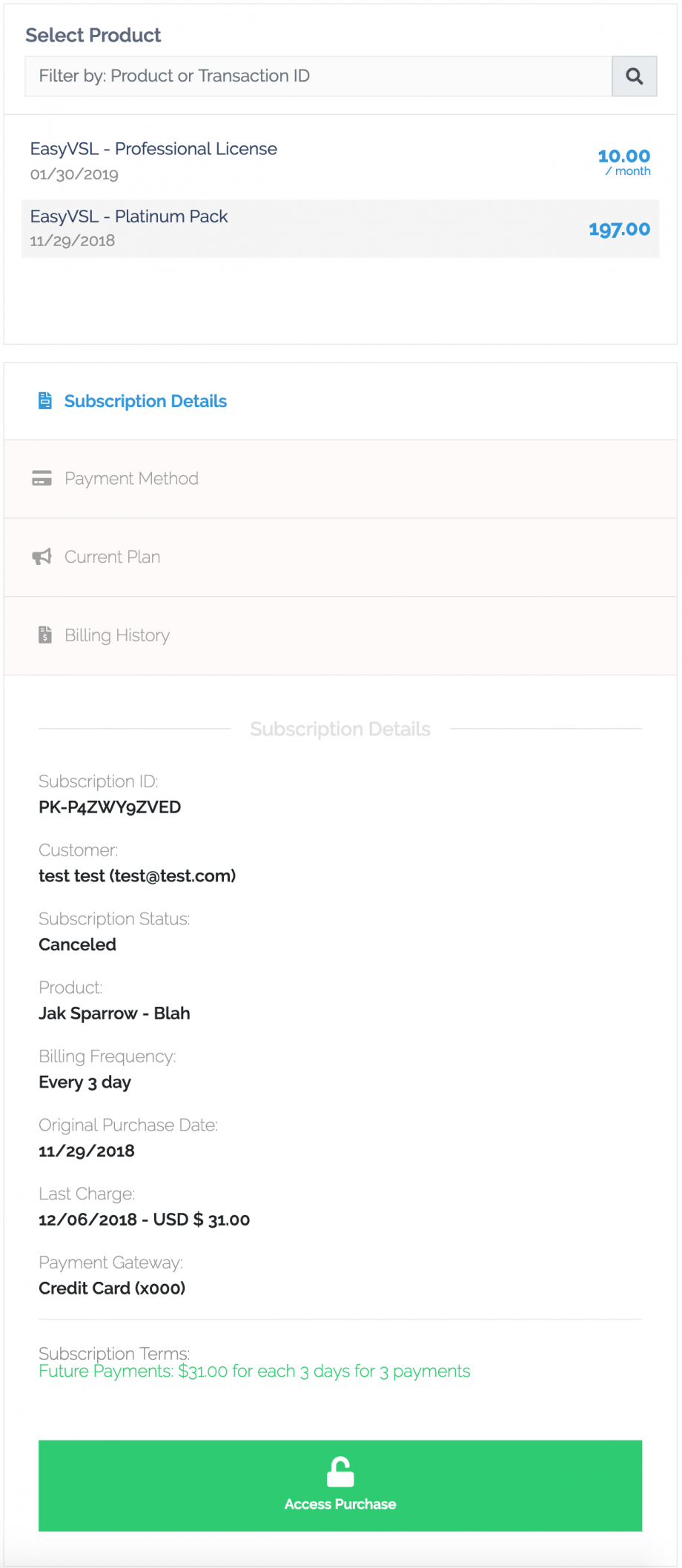The image features a user interface with a predominantly white background. At the very top, in bold black ink, is the title "Select Product". Below this title is a search bar with the placeholder text "Filter by product or transaction ID". To the right of the search bar, there is a magnifying glass icon indicating the search function.

Below the search section, two product descriptions are displayed in black ink. The first product, "EZVSL Professional License," includes the date "1-30-2019," and the price is listed as "$10 per month" in blue ink. The second product, "EZVSL Premium Pack," includes a date range depicting its validity until 2025, along with the price "$197" also in blue ink. Both prices and subscription details are prominently written in blue.

Farther down the image, the section labeled "Subscription Details" stands out in blue text. Below this heading are several categories in standard black or gray ink: "Payment Method," "Current Plan," and "Billing History". Below these categories, more specific information is provided under "Subscription Details". 

The subscription ID, listed as "PKPZWYGZVED," comprises mostly capital letters. The "Customer" field displays "test, test, test.com, or test, test, test at test.com." The "Subscription Status" is marked as "Canceled," and the "Product" is named "Jack Sparrow, blah." The "Payment Frequency" is stated as "Every three days," with the original purchase date noted as "11-29-2018" and the last charge date as "12-8-18," amounting to "USD $31." The payment type is indicated as "Credit Card."

A section labeled "Subscription Terms" provides further details. At the bottom of the description, there is a note about "Future Payment" of "$31 for three days for three payments," written in green text. Below this note is a green boxed area with a white lock symbol and the phrase "Access Purchase" written in white, signifying a secure payment access point.